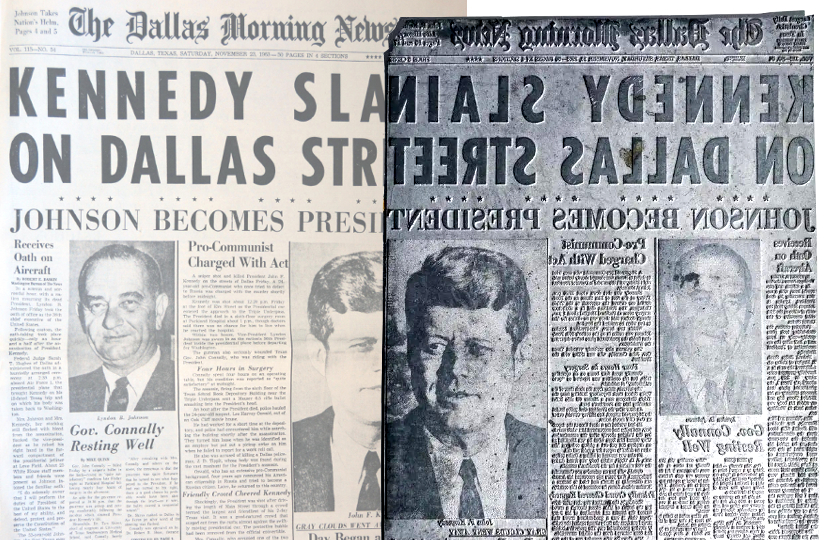The image is divided into two sides: on the left is a yellowed copy of an old newspaper from the 1960s, the Dallas Morning News, featuring a historic headline, "Kennedy Slain on Dallas Street," with a subheading, "Johnson Becomes President." This side of the image showcases a large, detailed article covering the assassination of John F. Kennedy and Lyndon B. Johnson's subsequent rise to the presidency. Prominently displayed are photographs of Kennedy on the left and Johnson on the right, surrounded by columns of text.

On the right side of the image, the newspaper's image is flipped and appears in a metallic, black-and-white negative form, showing the same pictures and text but in reverse, with raised metal print giving it a distinctive texture. The contrast is heightened, making the details of the reversed text and images sharp, stark, and visually striking. This inverted side highlights the physical metal form likely used to print the newspaper, illustrating the production process of the time.